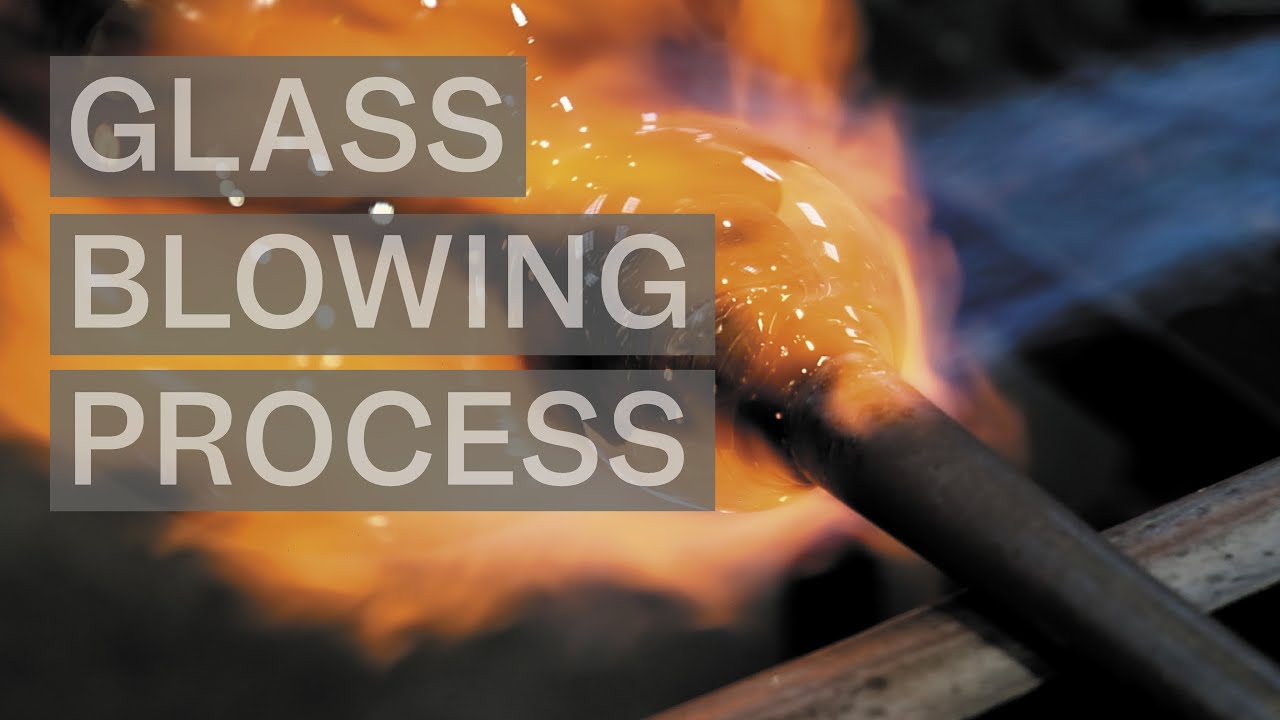The image depicts a professional-looking ad print with an ivory or off-white color scheme and large, uppercase letters positioned in the upper left corner, each word on a separate line. The text reads "GLASS BLOWING PROCESS" and is rendered in a see-through, oblique style, allowing the bright flames in the background to be partially visible through the letters. The background is predominantly black, highlighting the vivid flames surrounding a glowing, orange molten glass at the end of a metal rod, which enters the frame from the bottom left corner. The flames envelop the end of the rod, flowing towards the upper left section of the image.